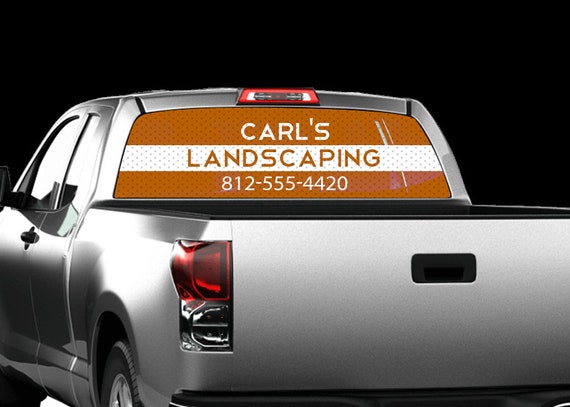This horizontal rectangular image features the rear of a shiny, silver pickup truck which appears to be new. The truck is set against a solid black background, enhancing its gleam. We can see the gate of the truck is closed, with a little black handle for opening it. The back window is adorned with an advertisement, which is a brown graphic wrap. The top strip of the wrap in white text reads "CARL'S," followed by a middle white horizontal stripe with "landscaping" written in brown letters, and a bottom brown strip with the phone number "812-555-4420" in white text. The image also reveals part of the driver's side of the truck, including the top of one tire, the side windows, and the tail light. The truck has a black tough shell lining in the bed area, suggesting durability. Overall, the image captures the sleek, pristine look of the pickup truck while clearly displaying the advertisement for Carl's Landscaping.